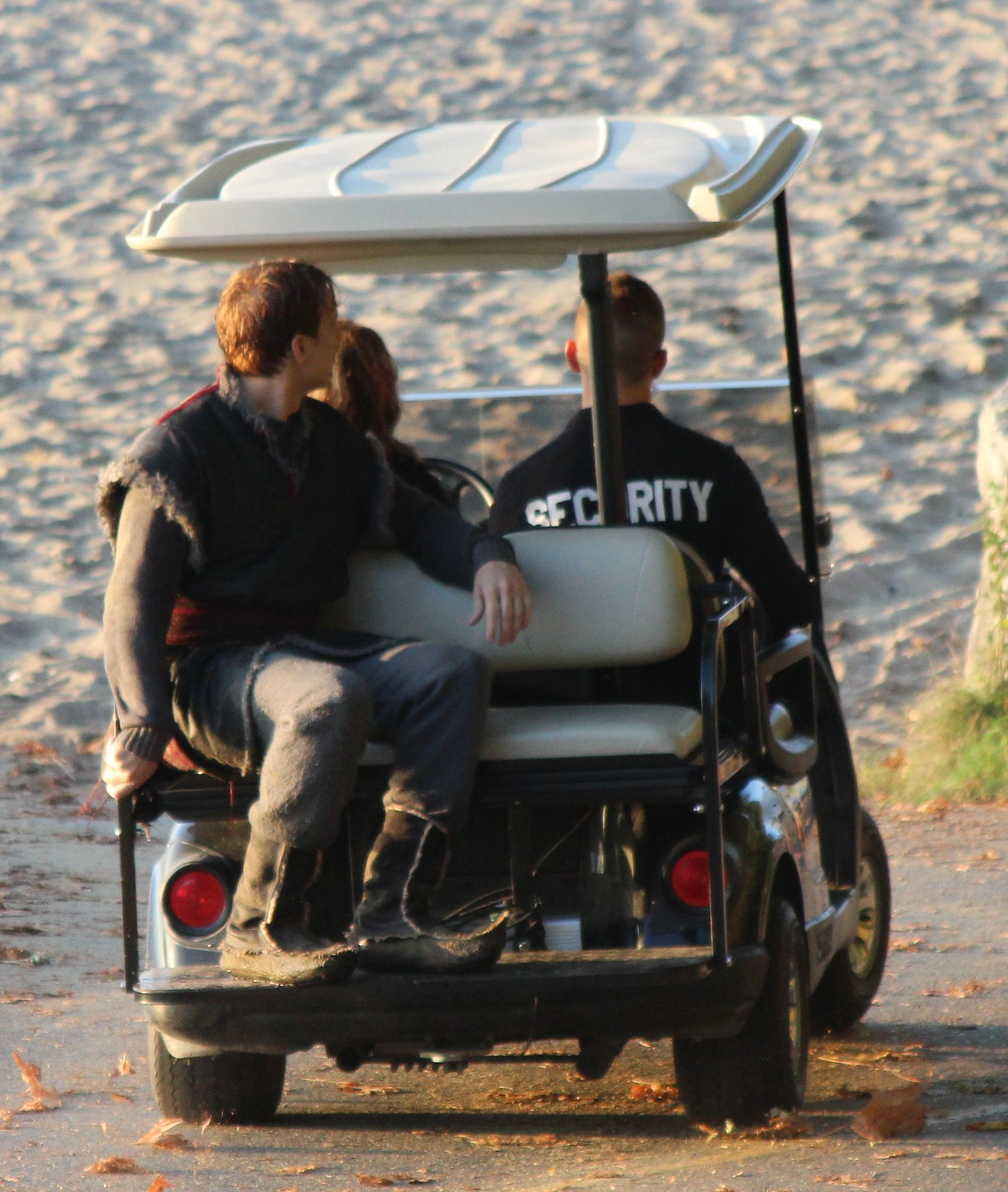This outdoor photo captures a golf cart traveling on a paved path near a large sandy field, possibly a beach, during sunset. The image is taken from behind, showing the rear and side of the cart. The golf cart, which has a top covering, features three occupants. In the front, a person with longer hair, most likely a woman, is driving, while to her right sits a young man with short hair wearing a black shirt with "SECURITY" printed in white on the back. In the back seat, facing away but turning his head forward, is a young person dressed in a fur-lined vest over a long-sleeved sweater, fleece pants, and rugged leather boots with upturned tips. All three individuals appear to be Caucasian. The lighting suggests that the sun is either setting or about to set, casting a warm glow over the scene.